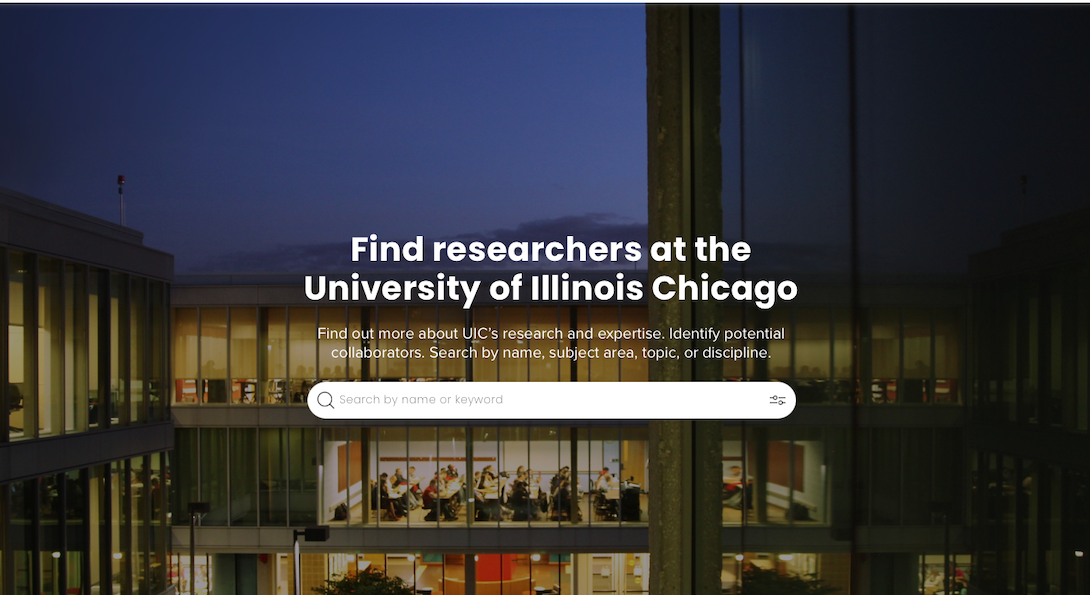The image features a rectangular layout with its longer side oriented horizontally. The backdrop showcases a U-shaped structure, resembling a single building extending on both sides and wrapping around to form an upside-down "U". This building, possibly part of an educational institution, consists of at least three visible stories with numerous windows that may indicate classrooms or offices.

On one of the levels, there is a group of people seated at tables, all facing the same direction towards a speaker or instructor positioned at the front, suggesting a lecture or presentation in progress. Above this scene, the sky is depicted with a dark blue hue and scattered high-altitude clouds, adding a serene atmosphere to the image.

Prominently displayed at the top of the building in bold, white text is the message: "Find researchers at the University of Illinois Chicago. Find out more about UIC's research and expertise. Identify potential collaborators. Search by name, subject area, topic, or discipline." Below this message, there is an elongated white search box with a search icon and the prompt, "Search by name or keyword."

This comprehensive view and informative overlay indicate a call to action for exploring research and collaboration opportunities at the University of Illinois Chicago.